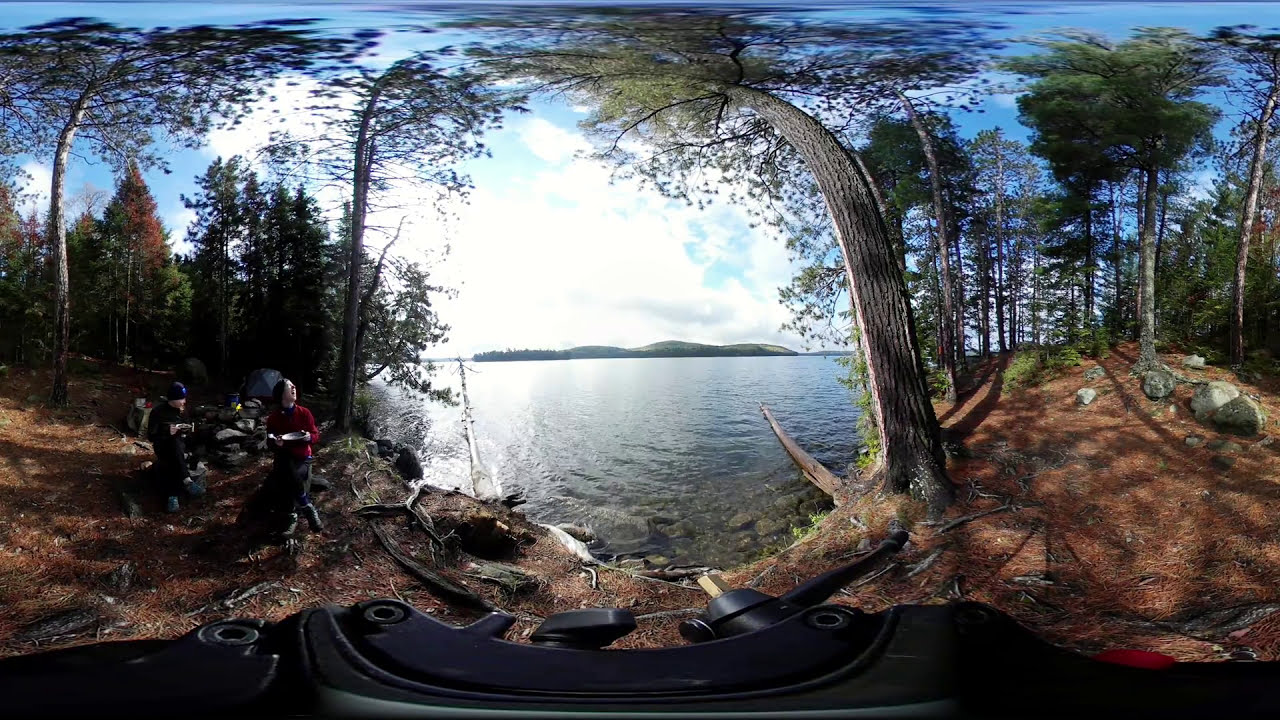Captured in a distorted, fish-eye view likely taken with a GoPro or VR setup, this image showcases an outdoor scene near a large, serene lake surrounded by a picturesque landscape. The lake, calm and reflective, sits at the center of the frame, under a sky that transitions from white to tinges of blue. In the foreground, the ground is a mix of brown dirt, sticks, and orange pine needles, typical of the Pacific Northwest environment. 

Two figures are prominent in the image: one wears a red jacket, black pants, and boots, while the other sports an all-black outfit with a black beanie and blue hiking shoes. They appear to be holding plates and are possibly seated or setting up a campsite, evidenced by the tents visible in the background. Towering pine trees, some bent and forming arches, frame the scene. There's an object at the bottom part of the image that resembles a black machine or possibly the dashboard of a vehicle. In the distance, a majestic mountain range stretches across the horizon, enhancing the scenic beauty of this unique, distorted photograph.